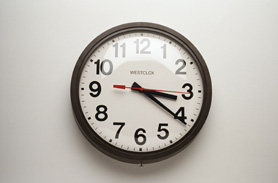The photograph features a simple, round analog clock mounted on a smooth, unadorned white wall. The clock has a dark housing, possibly brownish-black, framing a white face with bold black numbers ranging from 1 to 12. The clock's hands include long black rectangles for the hour and minute indicators, and a thin red second hand, which is currently positioned on the 3, marking roughly 20 seconds past the minute. The hour hand is on the 3 while the minute hand points to the 4, indicating the time is approximately 3:20. There is a shiny reflection on the glass or plastic protective cover over the clock face. Although slightly blurry, the clock's brand appears to be "West Clock."